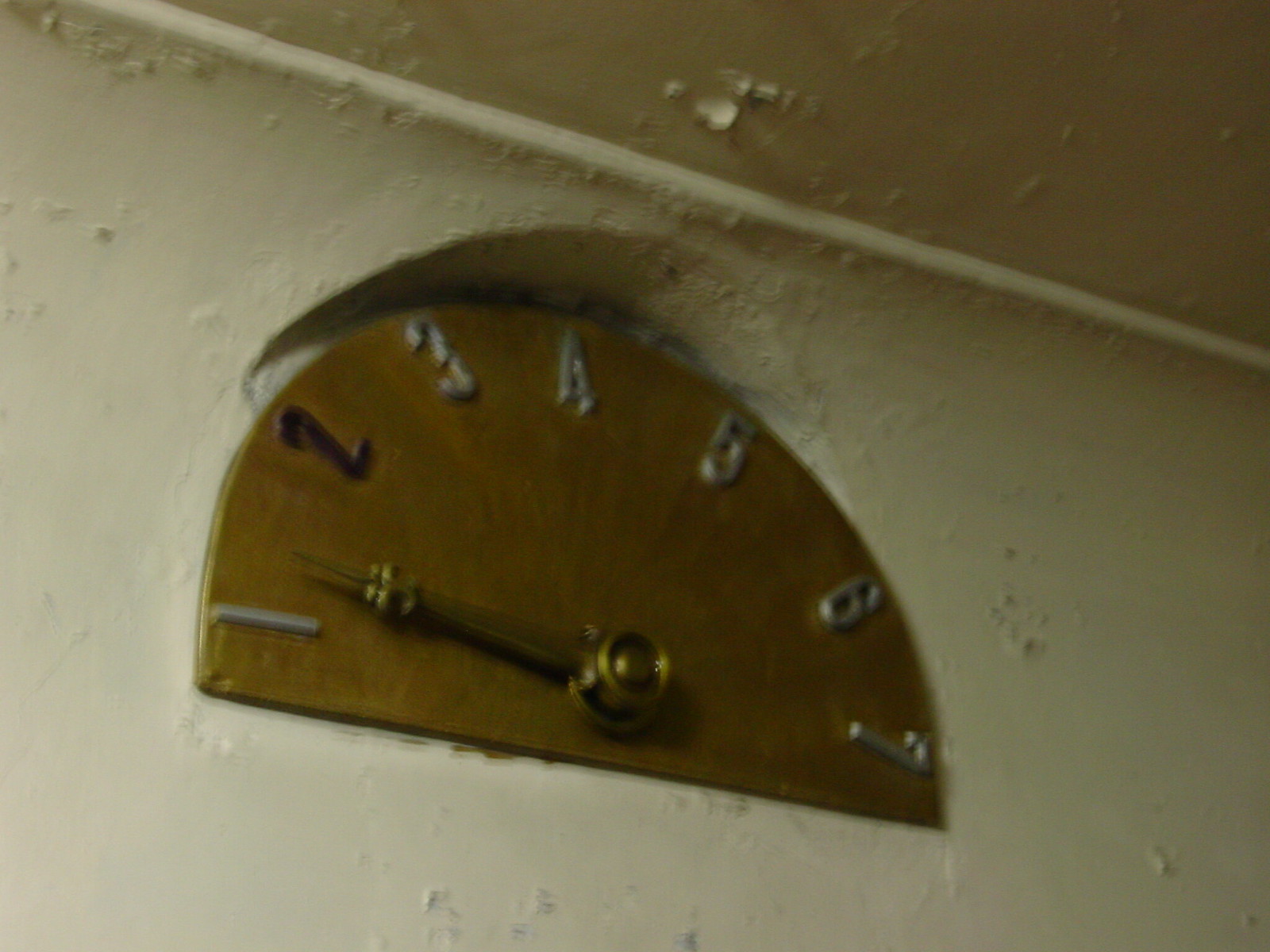This is a color photo depicting an old-fashioned elevator floor indicator, designed in a vintage half-circle style. The indicator, primarily composed of a golden bronze metal, features an arrow that resembles a clock hand, currently pointing to the first floor in the bottom left of the half-circle. The numbers on the indicator range from one to seven, with most in silver except for the number two, which is black. These numbers appear to be affixed to the surface of the plate. The device is slightly recessed into a white, stucco-like, plaster wall that is visibly aged, with several lumps, dust, and areas where the plaster is peeling, indicating its deteriorated condition. The ceiling above also shows signs of wear and peeling. The photo is framed in landscape mode, focusing on the upper section of the wall where the indicator is mounted.